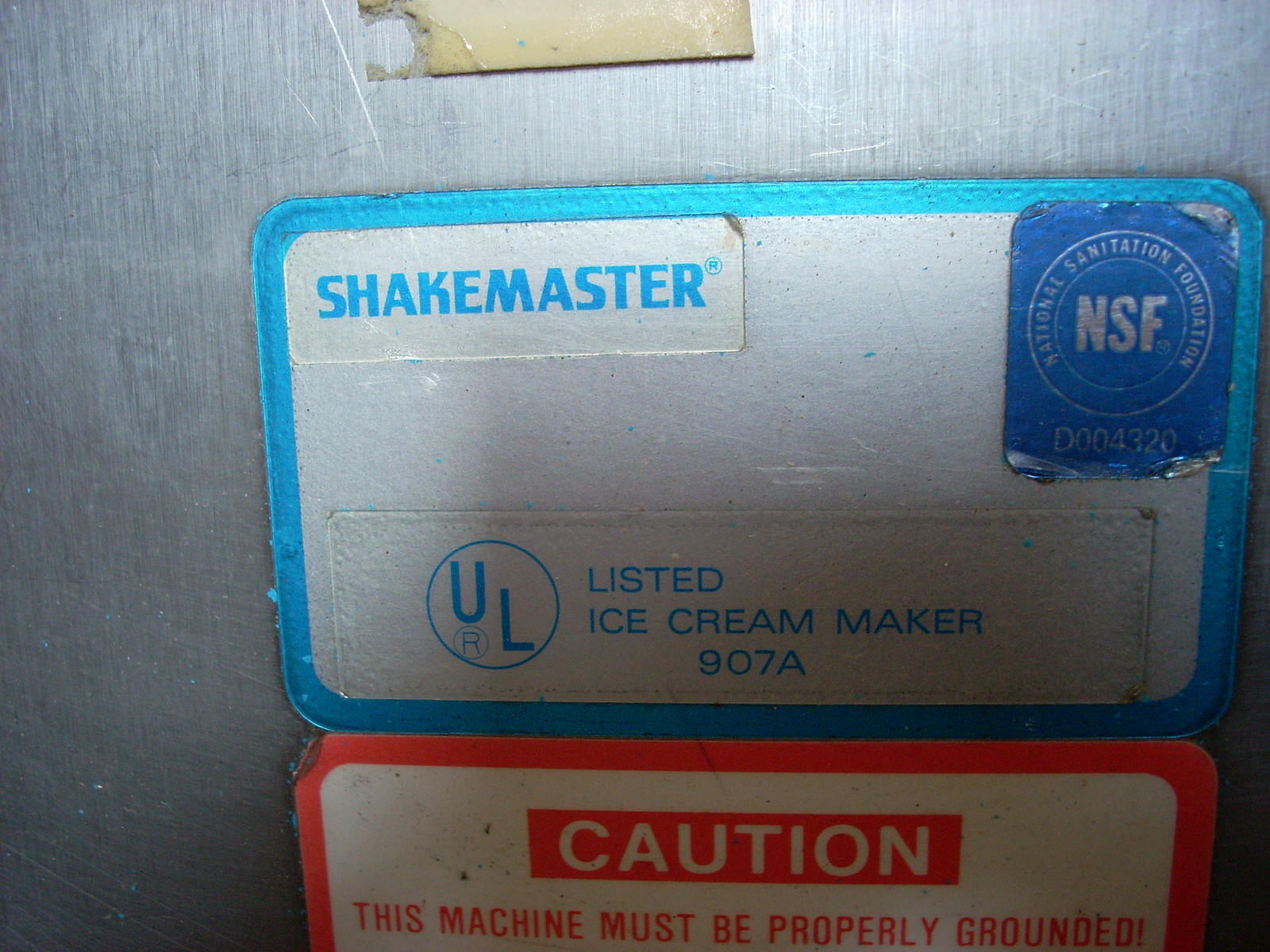This is an image of a metallic, presumably steel, surface which appears to be the side of an ice cream maker. The background is predominantly gray with some dark streaks and areas where the paint has peeled off. Prominently displayed are two labels. The top label is light gray with a rounded blue rectangle on the upper left that reads "Shakemaster". On the upper right, it has a blue circle with "NSF" inside, indicating certification by the National Sanitation Foundation. Text below this reads "UL Listed Ice Cream Maker 907A." Directly below this label is another light gray label with a red border. It displays a red caution box with white text stating, "This machine must be properly grounded." Additional text on this caution label is cut off in the image. The serial number "D004320" is also noted around the top label, though its exact position is not entirely clear within the image.